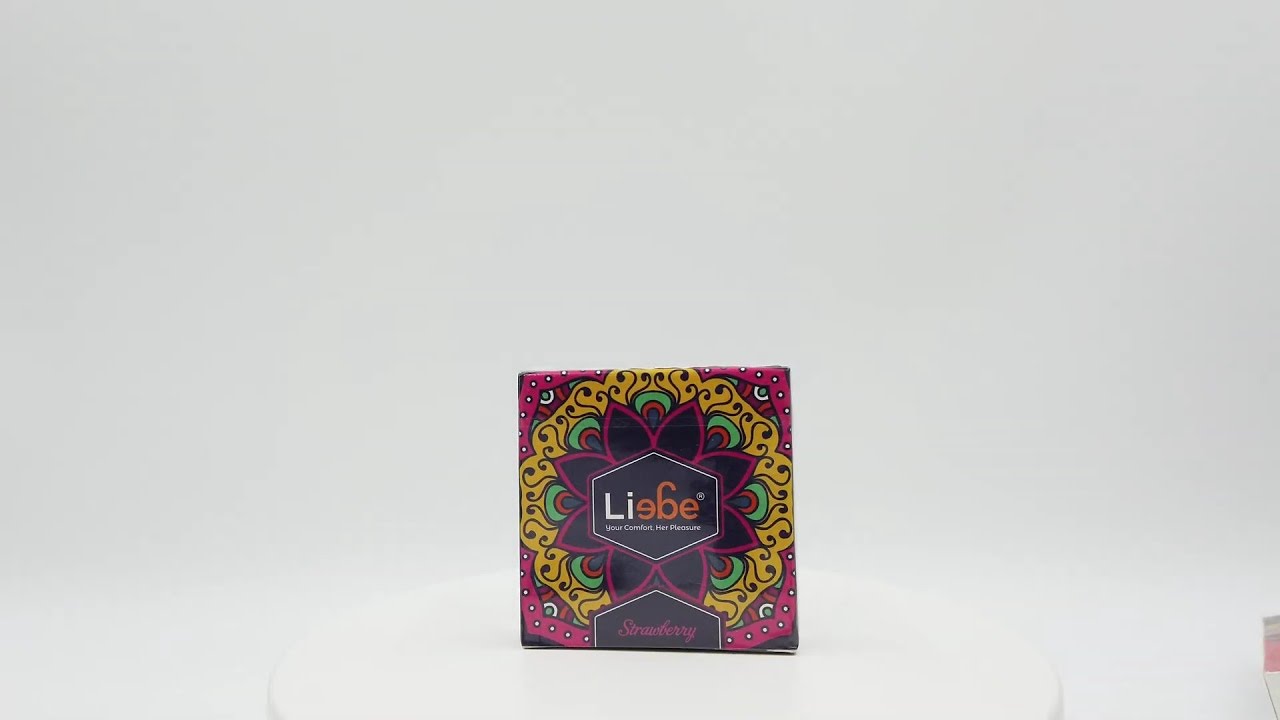The image depicts a highly detailed, photorealistic scene set against a flat white background. Centered near the bottom is a small, raised, almost indistinguishable, circular, white platform. Positioned on this platform is a small paper or box featuring intricate designs and text. Dominating the middle of this paper is a diamond shape outlined in white and further embellished with a pink border. Inside the diamond, the letters "L" and "I" are written in white, flanked by mirrored "E", "B", and "E" in orange. Below these letters, the phrase "your comfort, her pleasure" is inscribed in small white text.

Surrounding the diamond are vibrant flower and mandala patterns in pink, green, and gold, accentuated by white dots and black swirls. Each corner of the mandala is highlighted with dark reddish hues and dotted arches. A hexagon outlined in yellow with geometric shapes and plant-like strings intersects with these patterns. The bottom section of the paper features the word "strawberry" in pink cursive against a black background. Complementing the detailed designs, a partially visible cup with a see-through body capped in white adds a subtle contrast to the predominantly pink, green, and gold embellishments, enhancing the intricate and layered aesthetic of the image.